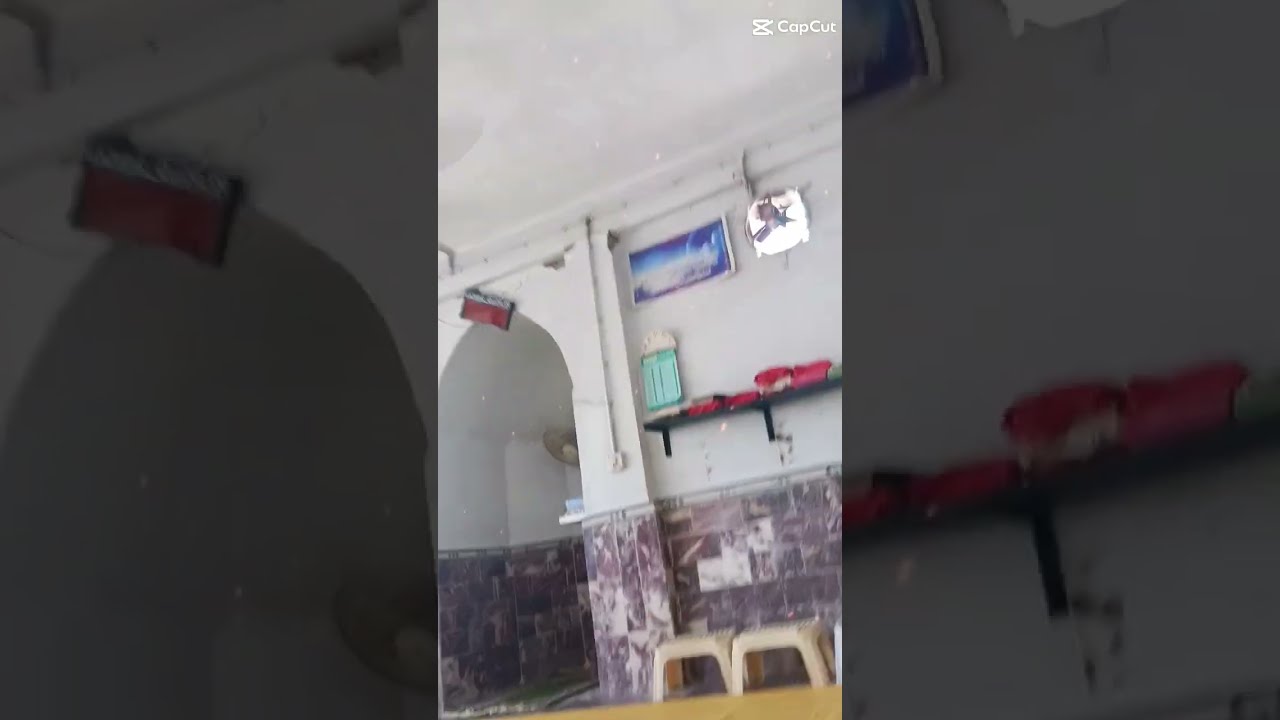This photograph depicts an old, worn room with distinct features suggesting it might be located in a third-world country. The upper portion of the walls are painted white, while the lower section consists of a purple and white tiled trim or possibly gray stone. The room is accessed through a large arched entryway. Attached to the wall is a black shelf holding red objects, with a turquoise square hanging above it. Above the square, there is a rectangular portrait that appears to depict a beach scene. The floor hosts two tan plastic footstools or benches positioned side-by-side. The overall impression of the room is one of disrepair, with peeling paint and a generally dilapidated appearance, and the photograph itself is slightly tilted counterclockwise. At the borders of the image, there are enlarged, grayed-out parts of the center scene, adding a unique framing to the photo. Additionally, wiring and electrics are visible within the room.